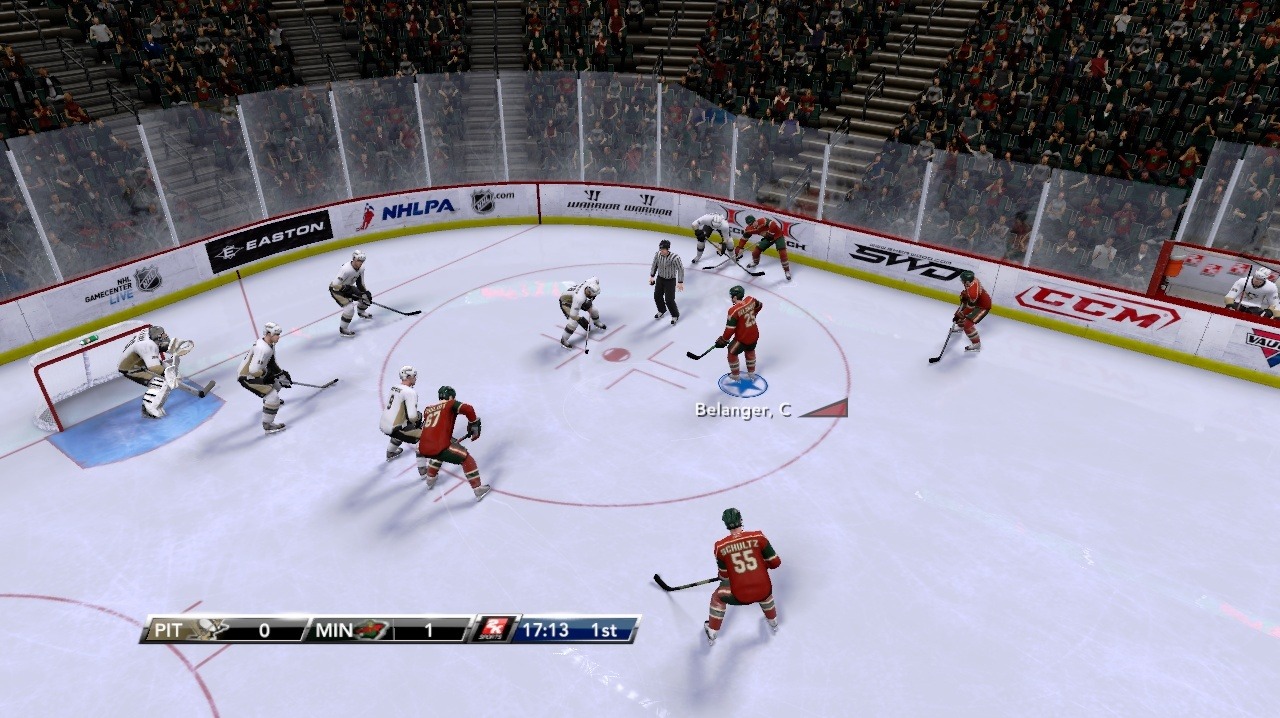The image depicts a repurposed hockey rink, once surrounded by ice. Advertising banners with brand names like Easton, H, LPA, SWD, and BCM are displayed prominently around the rink. Glass panels enclose the area, supported by white poles. The arena features multiple staircases and packed bleachers filled with spectators.

On the ice, players in both red and white uniforms are equipped with ice skates, hockey sticks, and helmets. A goalie stands guard in front of the net, ready to defend against incoming shots. The scoreboard displays the names "Pitt" and "2K," indicating team names or scores. The entire setup is unmistakably configured for an ice hockey game, capturing the intensity and excitement of the sport.